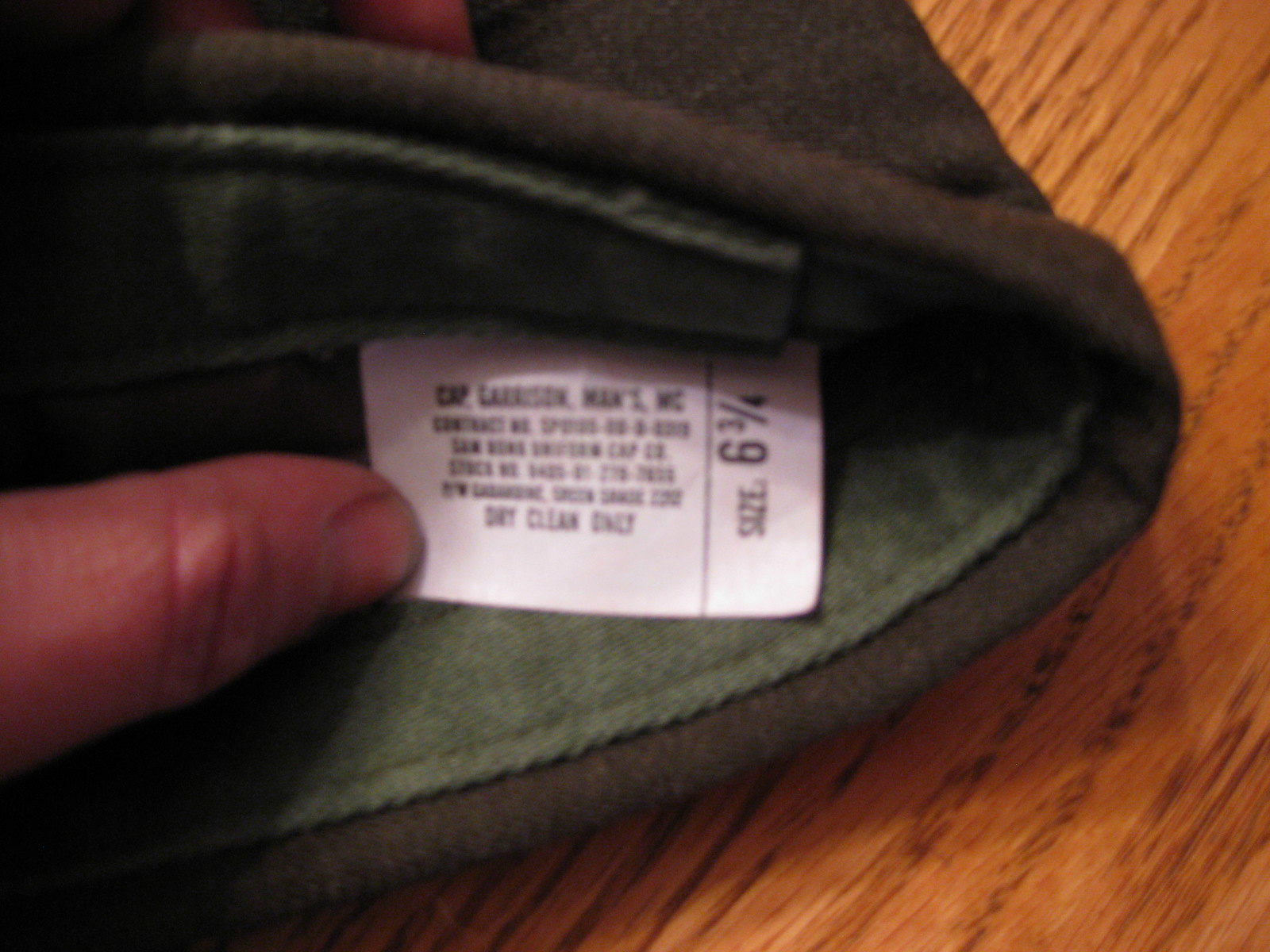The image displays a clothing tag affixed to a piece of fabric. Although some text on the tag is difficult to decipher, it appears to read "Kirsten Man" and "Small WC" on the left, and "Size 3.5" on the right. The tag also explicitly states that the item is "Dry Clean Only." The fabric, predominantly hunter green, features darker, brownish-green hues. The texture indicates it's a type of cloth, though the image is highly zoomed in, making it challenging to identify precise details. A person's thumb and pointer finger are holding the tag, with their nails clearly visible. The background reveals a brown wooden table with noticeable grain patterns, adding texture and depth to the scene.